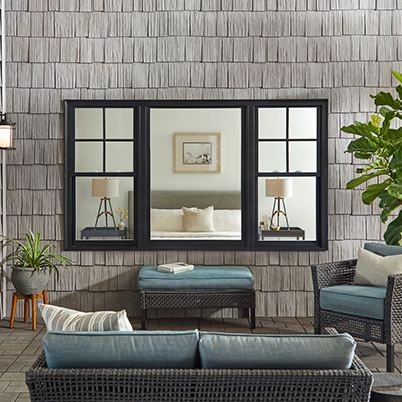This image showcases a stylish one-room studio apartment designed with careful attention to detail. The back wall is adorned with a realistic brown brick-patterned wallpaper, setting a warm, rustic tone. A multi-panel mirror with a distinctive four-pane top section hangs prominently, reflecting elements of the room to create an illusion of space. Beneath the mirror sits a plush blue ottoman, adding a splash of color and functionality.

To the left of the scene, a gray pot houses a vibrant potted plant, bringing a touch of greenery indoors, while the right side features a larger potted tree, contributing to a natural ambiance. A cozy chair with a blue cushion and a white pillow sits invitingly, complemented by a sofa, or loveseat, whose back is visible. This sofa is adorned with blue and white pillows, tying the color scheme together.

Interestingly, the mirror reflects the image of a neatly made bed, complete with a gray headboard, white pillows, sheets, and covers. This detail suggests that the space is multifunctional, likely serving as both a living and sleeping area typical of a studio apartment.

In the background, hints of the exterior are visible, with gray siding and a central window that lets in natural light. The reflection also offers glimpses of two nightstands, each with a lamp, hinting at a cozy and well-coordinated bedroom setup. Each of these elements comes together to create a cohesive, functional, and aesthetically pleasing living space that could very well be featured on a design or furniture site.